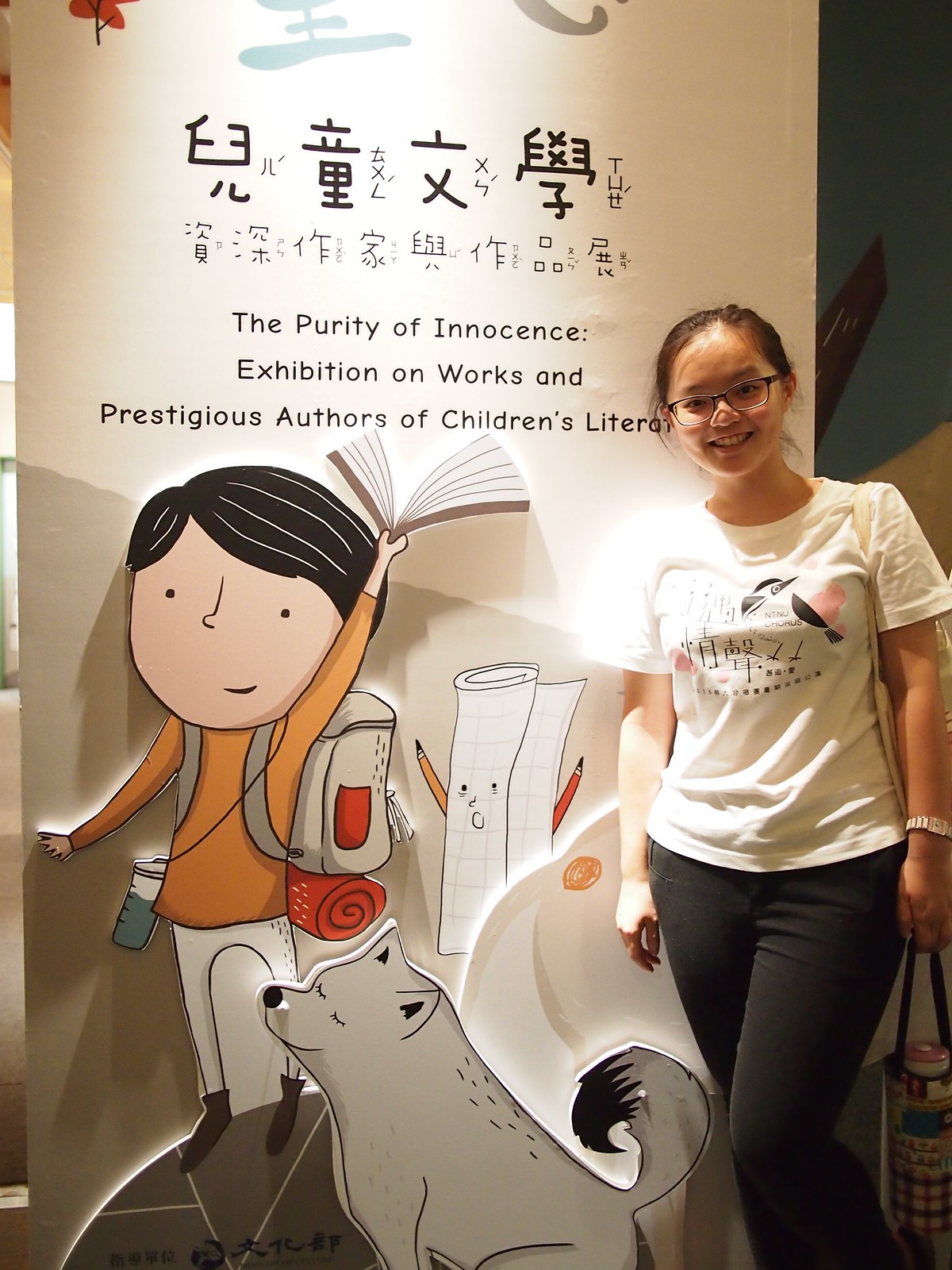In the image, a young Asian woman, possibly in her late teens or early 20s, is standing in front of a large, vertical banner with a cream-colored background, part of an art installation. She has tied-back hair, wears glasses, a white t-shirt with Chinese text and a small bird illustration, black pants, and carries a canvas bag over her shoulder along with a water bottle. A white wristwatch adorns her left wrist. The banner she's standing in front of features colorful designs and Chinese text at the top, with an English translation below that reads, "The Purity of Innocence: Exhibition on Works and Prestigious Authors of Children's Literature."

The lower portion of the banner displays an animated scene depicting a young schoolboy wearing an orange shirt and gray backpack with a red pocket, white pants, and black boots. He is holding an open book and has a water bottle strapped around his side. Standing near his knees is a small dog, possibly a Shiba Inu, and beside him is a roll of paper with a face, yellow and red pencils as arms, observing the boy. A spotlight shines on the scene, casting a reflection off the girl's shoulder and the backdrop. The setting is within a building, though the specific location remains unclear.